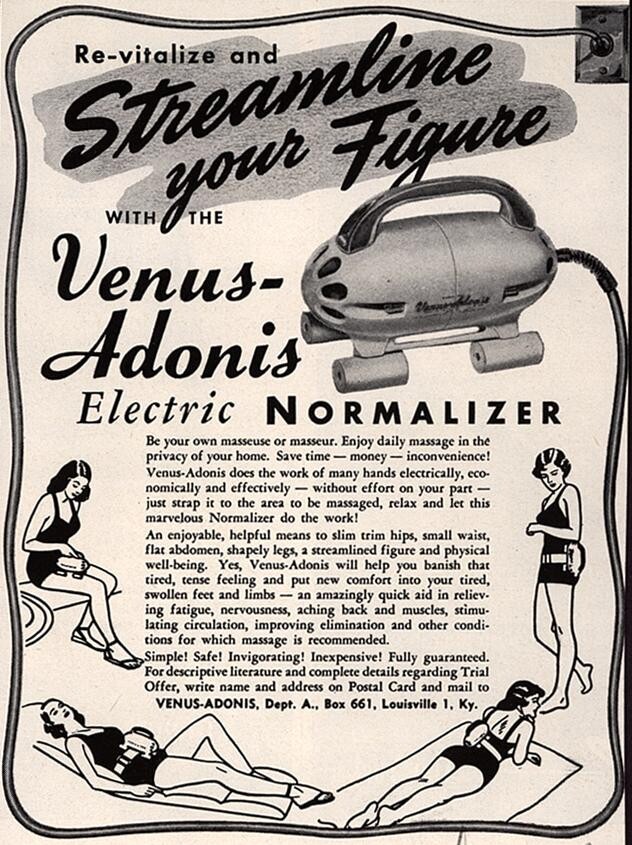This vintage black and white advertisement spotlights the "Venus Adonis Electric Normaliser," designed to rejuvenate and streamline the user's figure. The background is a creamy off-white, with the ad framed by a grayish black-outlined border, emphasizing an old-fashioned aesthetic. Dominating the top in prominent black text, the headline reads, "Revitalize and streamline your figure," with "streamline your figure" artistically rendered in cursive against a subtle gray backdrop. Below, it introduces the product name, Venus Adonis, and a detailed paragraph extolls its virtues: "Be your own masseuse or masseur. Enjoy daily massages in the privacy of your home. Save time, money, and inconvenience..."

This transformative massager, depicted with a bullet-shaped main body and black handle, promises to mimic the efforts of many hands electrically, economically, and effectively, all while strapped comfortably to the targeted area. Four cartoon-style illustrations of women in bathing suits showcase its usage on various body parts like the stomach, back, and sides, underlining its target market of young women looking to achieve slimming and toning results. The text highlights its numerous benefits including alleviating fatigue, promoting circulation, and relieving muscle aches, all while being simple, safe, invigorating, and inexpensive. For further details and a trial offer, prospective buyers are invited to contact Venus Adonis, adding a personal touch to this nostalgic piece of fitness marketing.